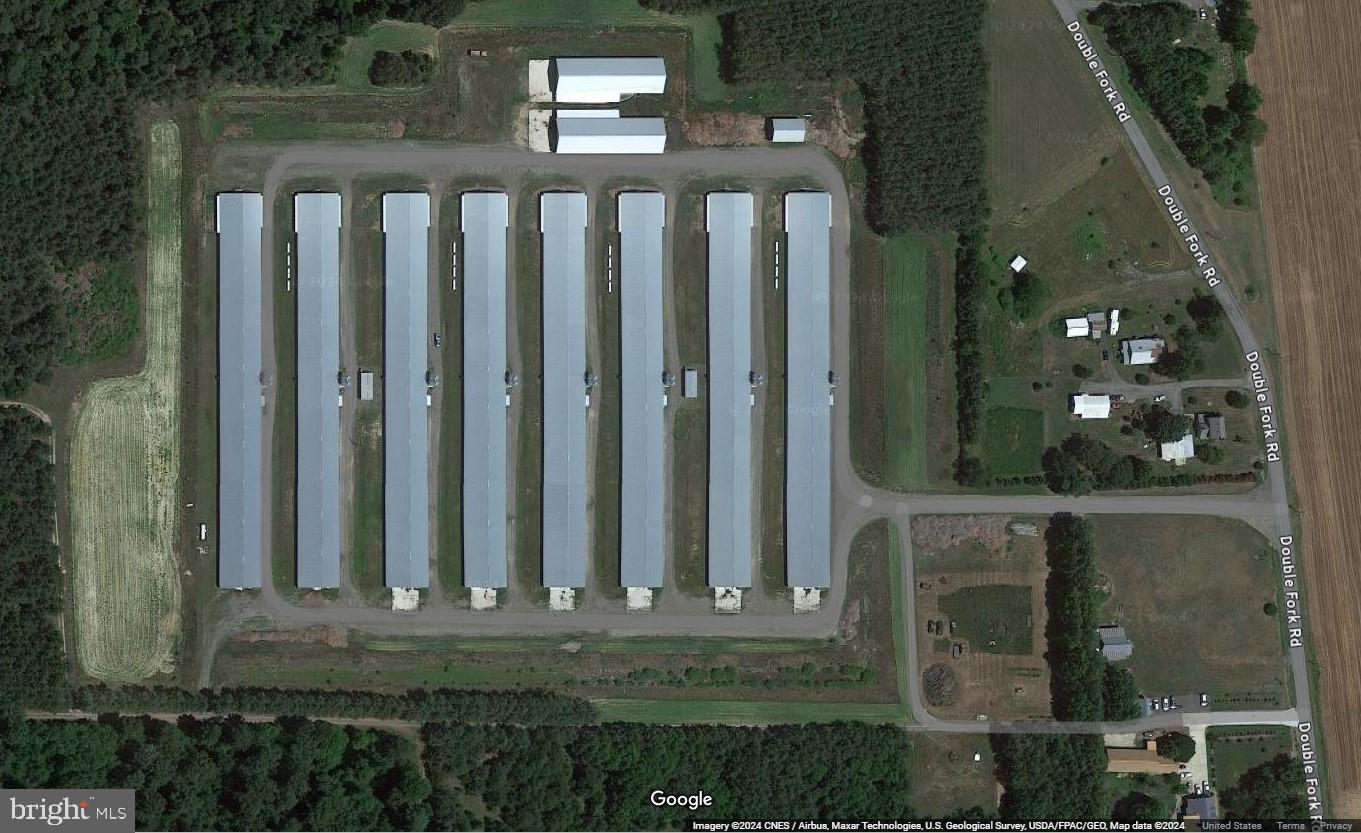This aerial view image, labeled with “BrightMLS” in the bottom corner and sourced from “Google Imagery 2024 CNS Airbus Master Technologies U.S. Geology Survey,” showcases a rural area dominated by eight long, gray metal buildings. Situated near the center-left of the image, these buildings are distinctly rectangular and aligned in parallel rows, each approximately 20 times the length of the smaller surrounding structures. 

The right-hand side of the image is bordered by Double Fork Road, from which two smaller roads branch off to connect to the complex of large buildings. These roads also lead to smaller areas with clusters of smaller buildings and houses, including one cluster of five and another of three houses. The scene is framed by dense green foliage indicative of a forested area, while the immediate vicinity of the large buildings features well-maintained lawns and additional smaller roads.

The purpose of the long buildings is unclear, possibly suggesting uses ranging from storage units to, more speculatively, a military installation, as no detailed markers or people are visible from this aerial perspective. Small outbuildings and sporadically parked cars are also present, contributing to the sense of an organized but somewhat enigmatic site amid a predominantly green, rural landscape.